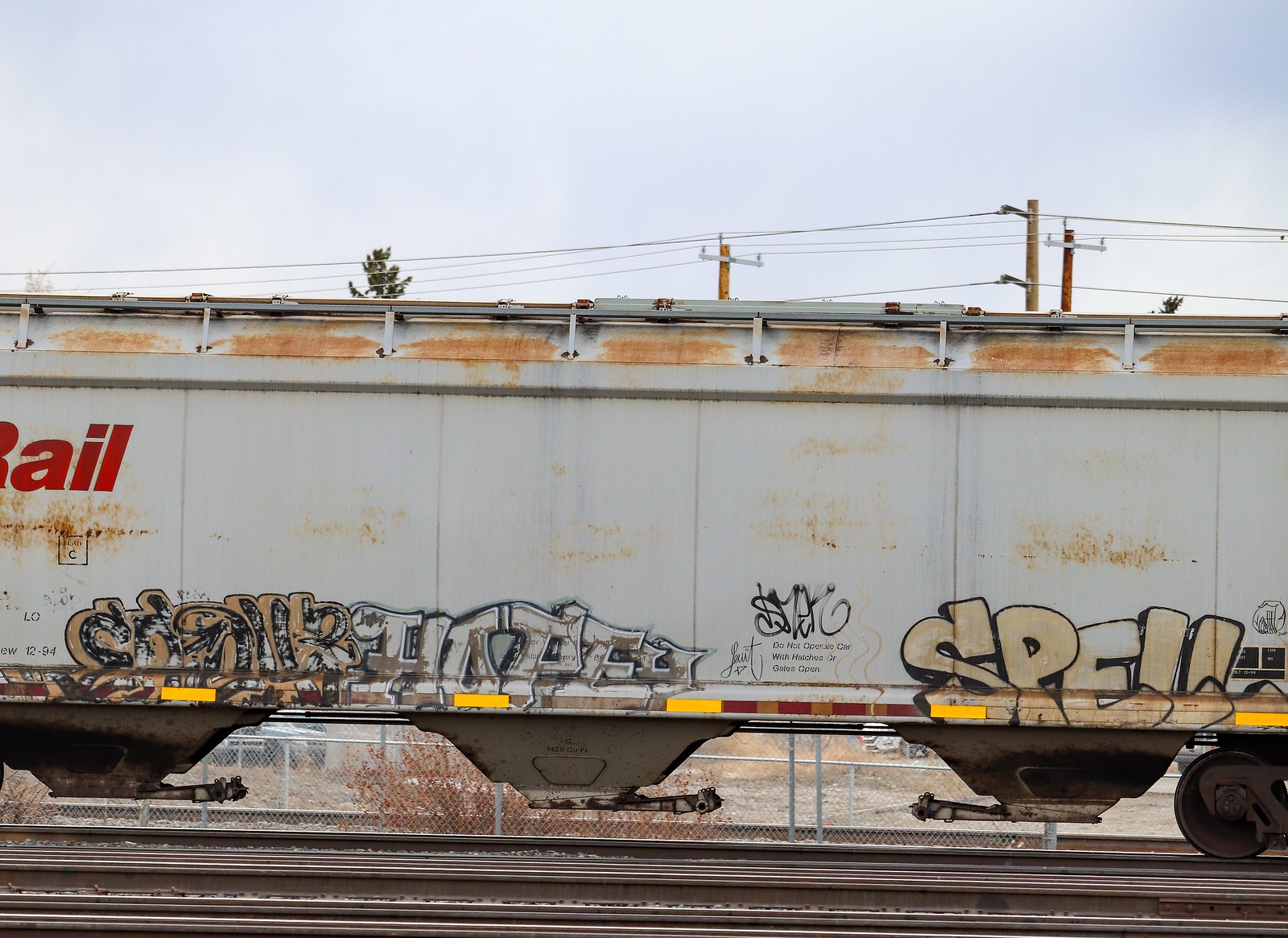The photograph depicts a partially visible white railroad car situated outdoors on a railroad track. The sky, while slightly overcast, still allows for a bright ambiance, accentuated by the presence of some clouds. The train car exhibits significant rust, particularly along the upper and lower portions, contributing to its weathered appearance. Prominent graffiti adorns the car, with the word "SPELL" in tan lettering clearly visible on the lower right-hand side. Adjacent to this, other tags in black and tan have been applied, though they are less distinct. On the upper left-hand corner, the word "RAIL" is boldly inscribed in red letters. Behind the car, tall utility poles and part of a tree are noticeable, adding depth to the scene. Below the car, the wheels and some underlying fence are also visible. The image captures a singular section of the train car, emphasizing the blend of decay, utility, and urban art.